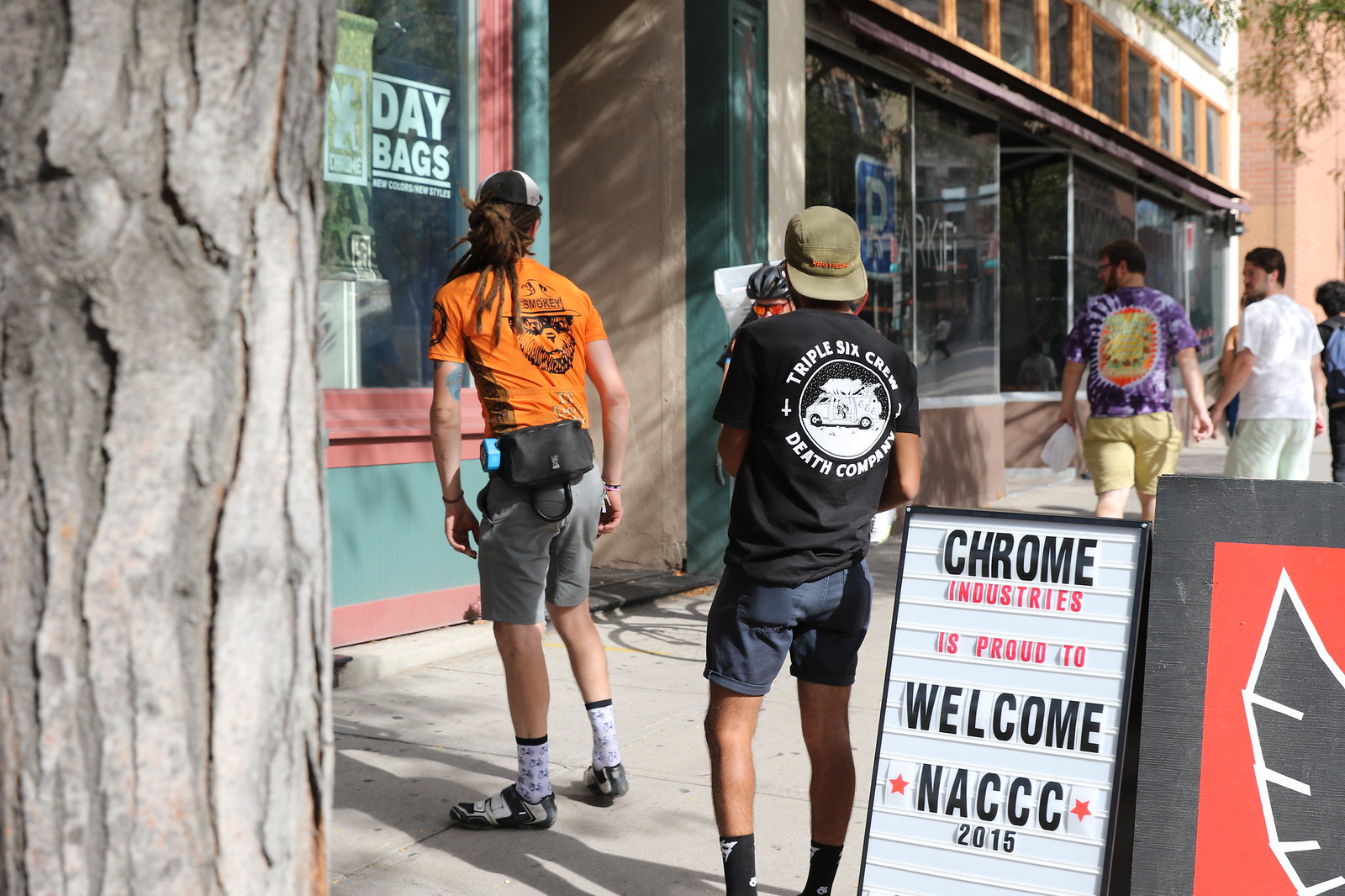In this horizontal landscape photograph, a diverse group of people are on a sidewalk framed by a large tree on the far left that stretches vertically from the bottom to the top of the image. The closest to the camera is a person in an orange t-shirt, featuring black illustrations, possibly resembling Smokey Bear, paired with gray shorts and athletic shoes that look like climbing shoes. This individual sports a fanny pack, a hat, and has dreadlocks. Positioned behind them is another person clad in a black t-shirt with white writing and a graphic of a van within a circle, labeled "Triple Six Crew Death Company." This second person is also wearing blue shorts, black socks, and a green five-panel hat worn backward. They seem to be holding something in front of their face, possibly a paper.

Further down the sidewalk, two men walk hand in hand. One is dressed in a white t-shirt and mint green shorts, while the other wears khaki shorts with a purple tie-dye shirt. Both are strolling past storefronts, one of which prominently features a white sandwich board sign that reads, "Chrome Industries is proud to welcome NACCC 2015," with adjacent indistinct signage that appears to show black wings above a red square on a black background. In the background, the sidewalk extends to reveal more storefronts and the partial view of another building's corner, completing the bustling urban scene.